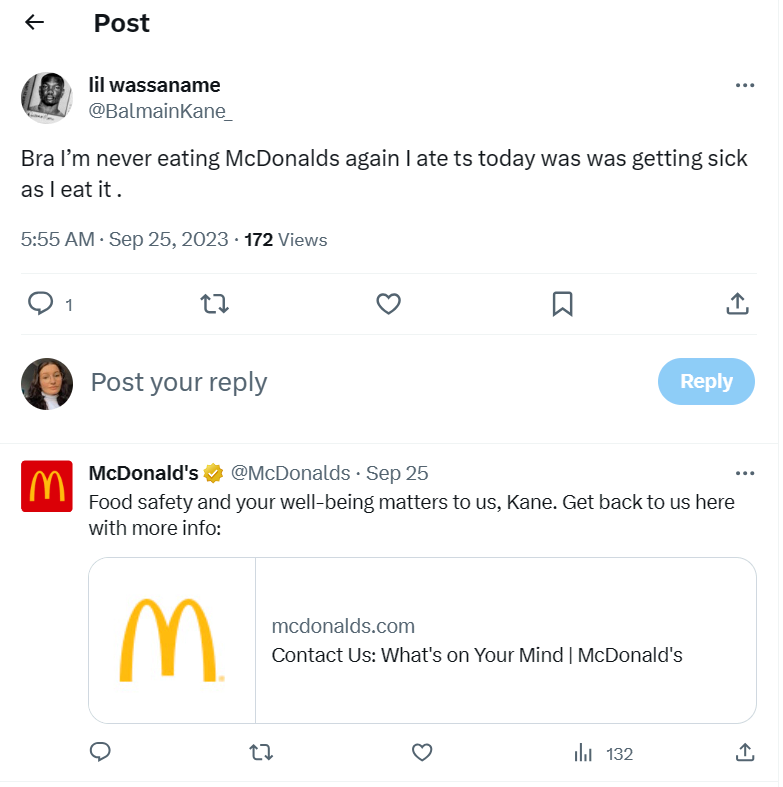The image depicts a detailed post from a website featuring a minimalist white backdrop with black writing, unless otherwise stated. 

**Layout and Header:**
- **Top Left Corner:** A black arrow pointing to the left.
- **Next to the Arrow:** A bold black text stating "Post."
- **Remainder of the Top:** Blank.

**User Information:**
- **Bottom Left Corner below the Header:** A circular avatar featuring a black man with a beard and mustache.
- **To the Right of the Avatar:**
  - **Username:** "Lil Wassaname" (L-I-L W-A-S-S-A-N-A-M-E).
  - **User Handle:** "@BalmainKane_" with B and K capitalized.

**Post Content:**
- **Body of the Post:** "Bruh, I'm never eating McDonald's again. Ate T-S today, was getting sick as I eat it."
- **Timestamp:** "5, 5:55 a.m., Sep 25, 2023, 172 views."
- **Interaction Icons and Counts:** 
  - Speech bubble with the number 1 (comments),
  - Retweet symbol,
  - Heart icon,
  - Ribbon icon,
  - Save icon.

**Reply Section:**
- **Reply Avatar:** A circle with a Caucasian woman with brown hair in a white turtleneck and black blazer.
- **Text:** "Post your reply."
- **Reply Button:** A blue bar with white text reading "Reply."

**Brand Response:**
- **Red Box with Yellow M:** McDonald's logo.
- **Text:** "McDonald's @ McDonalds. SEP25. Food safety and your well-being matter to us, Kane. Get back to us here with more info."
- **Link Section:**  
  - Yellow McDonald’s Golden Arches logo,
  - Text: "McDonalds.com, Contact us, What's on your mind / McDonald's."

**Bottom Interaction Icons:**
- **Icons with Counts:** 
  - Comment icon (speech bubble),
  - Retweet logo,
  - Heart logo,
  - Four black lines, 
  - "132" next to the save icon.

This composition captures the layout and detailed elements in the image, reflecting a structured interaction post reminiscent of social media platforms.